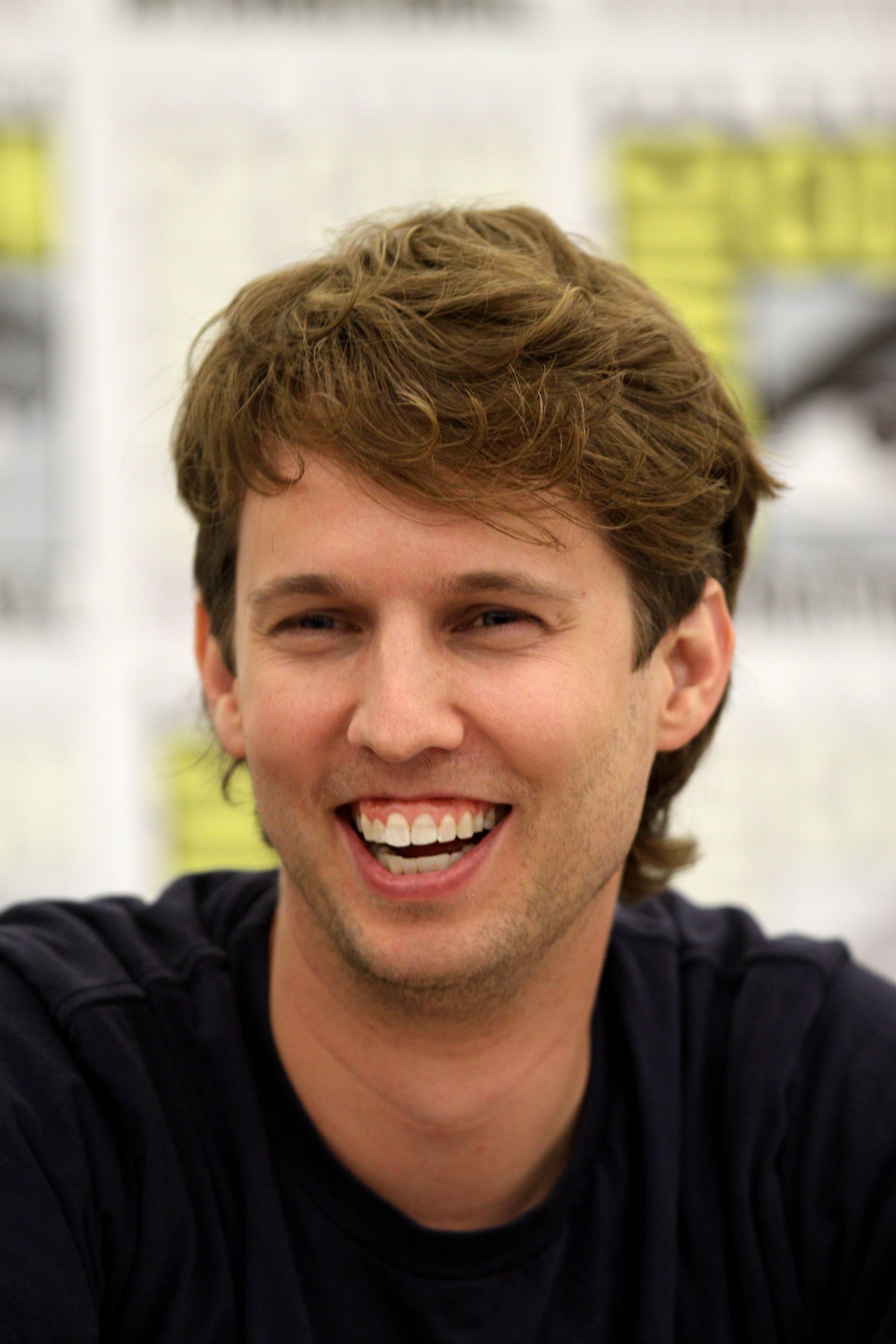This is a portrait-oriented photograph featuring a smiling Jon Heder, famously known for his role in "Napoleon Dynamite." The image, which captures Jon from his shoulders upwards, showcases him in the foreground with a slightly off-camera gaze towards the left side of the frame. He sports a black crew neck t-shirt and has shoulder-length, light brown hair styled in a casual mullet. His face displays a full-toothed smile, revealing both the top and bottom rows of his teeth, along with dark-colored stubble on his cheeks and chin. In the background is a slightly blurry whiteboard adorned with a repeating Comic-Con logo in yellow text, interspersed with giant eyeball icons, suggesting the photo was taken at a Comic-Con event. The whiteboard provides a recognizable yet out-of-focus backdrop, emphasizing Jon Heder's cheerful and relaxed demeanor in the close-up shot.